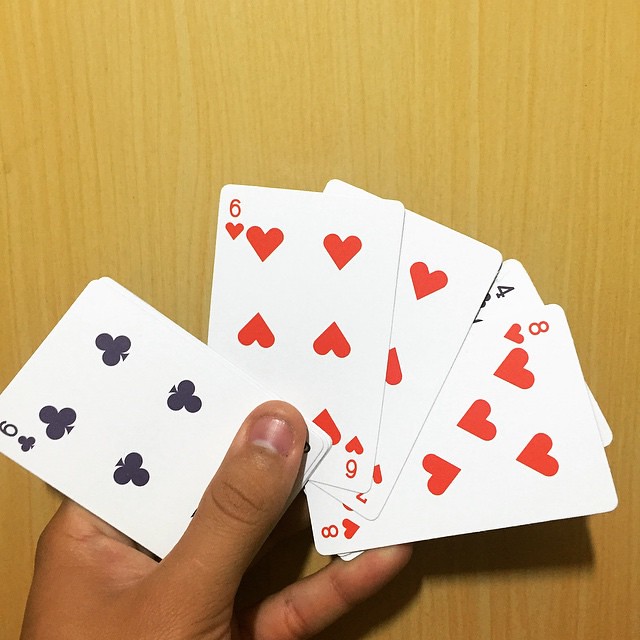In this photograph, a person with a medium-dark brown complexion and neatly trimmed short nails holds a fan of playing cards against a light wooden table. The visible cards include a six of clubs, a six of hearts, a partially hidden seven of hearts, an eight of hearts, and a four of clubs. The cards are spread loosely, with some clumped together, making it difficult to discern the exact number, though there appear to be at least seven in total. The lighting casts shadows of the cards onto the table, suggesting the presence of artificial illumination. The individual seems to be preparing for a card game, as indicated by the way the cards are arranged and held.